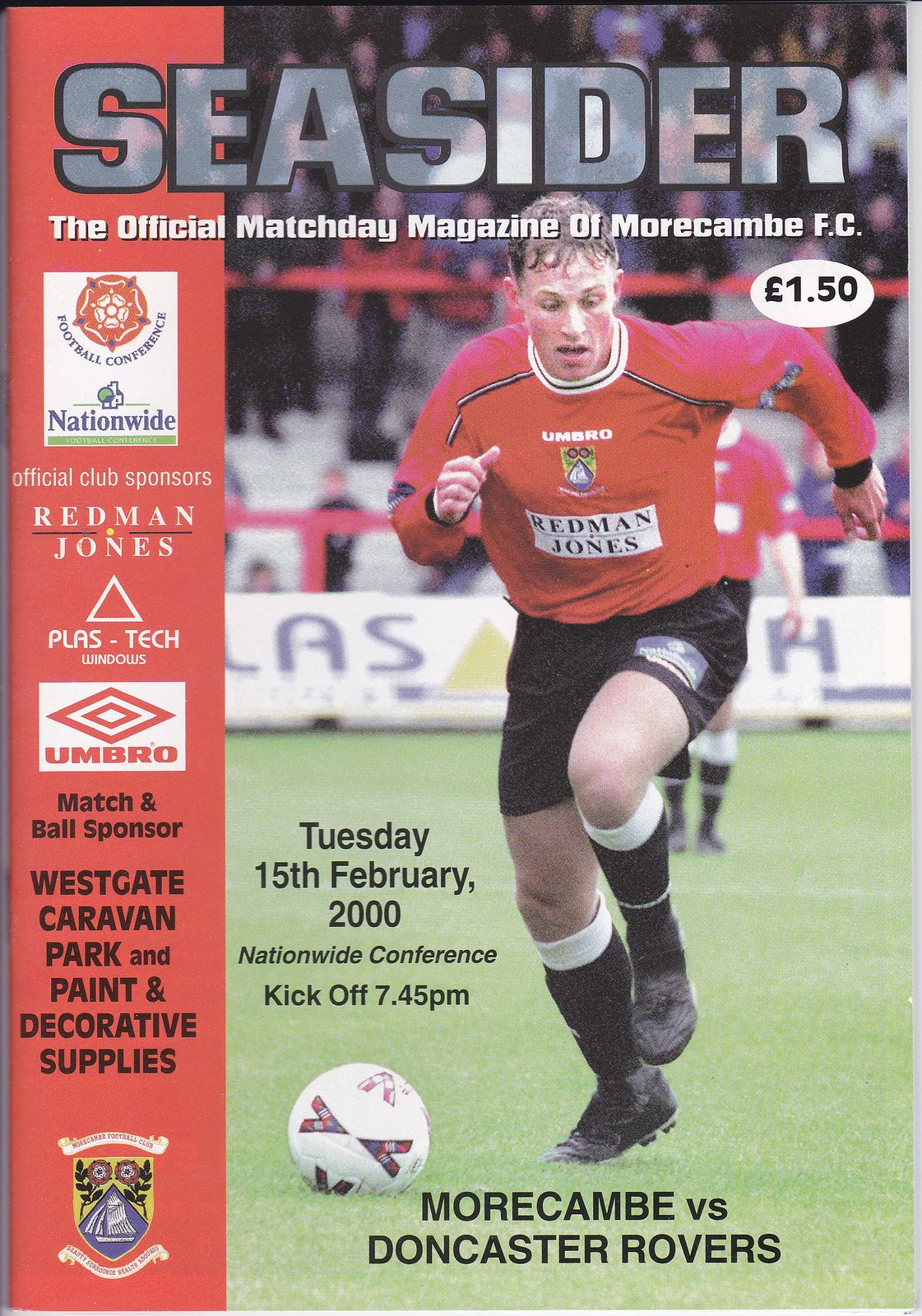The image depicts the cover of a 2000 edition of an English football club program, titled "Seasider," which is the official match day magazine of Morecambe F.C. At the top, in gray, it reads "Seasider," with "The official match day magazine of Morecambe F.C." written in white below. Within a white oval, it states "£1.50" in black. 

Central to the cover is an action shot of a player, who is a Caucasian man with light, sweaty, matted-down hair. He is captured in mid-action, playing soccer, and appears to be running towards the camera. He is outfitted in a long-sleeved red jersey with "Redmond Jones" printed on it, black shorts, black socks, and black shoes. 

Behind him, a crowd of spectators is visible but blurred to emphasize the player's movement. To the left of the player, text details the event: "Tuesday, 15th February 2000, Nationwide Conference, kickoff 7.45 p.m." At the bottom, it announces the match: "Morecambe versus Doncaster Rovers." Along the left edge, a red banner runs from top to bottom, featuring various logos and writings.

Additionally, sponsors of Morecambe F.C. are mentioned, including Redmond Jones, Plastic Windows, Umbro, Westgate Caravan Park, and Paint Decorative Supplies.